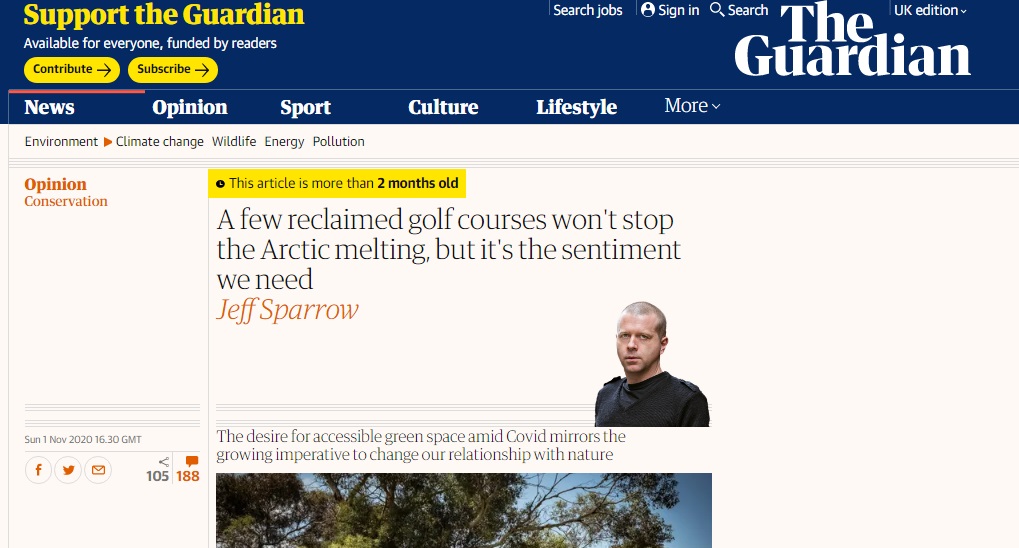The image depicts a webpage from The Guardian, featuring a prominent rectangular banner across the top. The banner is colored navy blue, with yellow accent text. On the upper left-hand side of the banner, text in yellow reads, "Support The Guardian," followed by "available for everyone, funded by readers." There are two clickable yellow buttons: the first one says "Contribute" and the second one, located beside the first, says "Subscribe," both in large white letters.

On the right side of the banner, options for user interaction are available, including "Search," "Sign in," and a job search feature. The version shown appears to be the UK edition of The Guardian.

Beneath this primary banner lies a secondary navigation bar featuring several tabs, arranged from left to right: "News," "Opinion," "Sport," "Culture," "Lifestyle," and a "More" dropdown menu. These tabs allow users to navigate to their desired sections of the website.

The article displayed is classified under the "Opinion" section and is focused on conservation efforts. Highlighted in yellow, an annotation alerts readers that the article is "more than two months old." The headline of the article reads, "A few reclaimed golf courses won't stop the Arctic melting but it’s the sentiment we need," authored by Jeff Sparrow. Accompanied by a picture of a man, the subheading states, "The desire for accessible green space amid COVID mirrors the growing imperative to change our relationship with nature."

The article was published on Sunday, November 1, 2020. At the time of capture, the article had accumulated 105 shares and 188 comments.